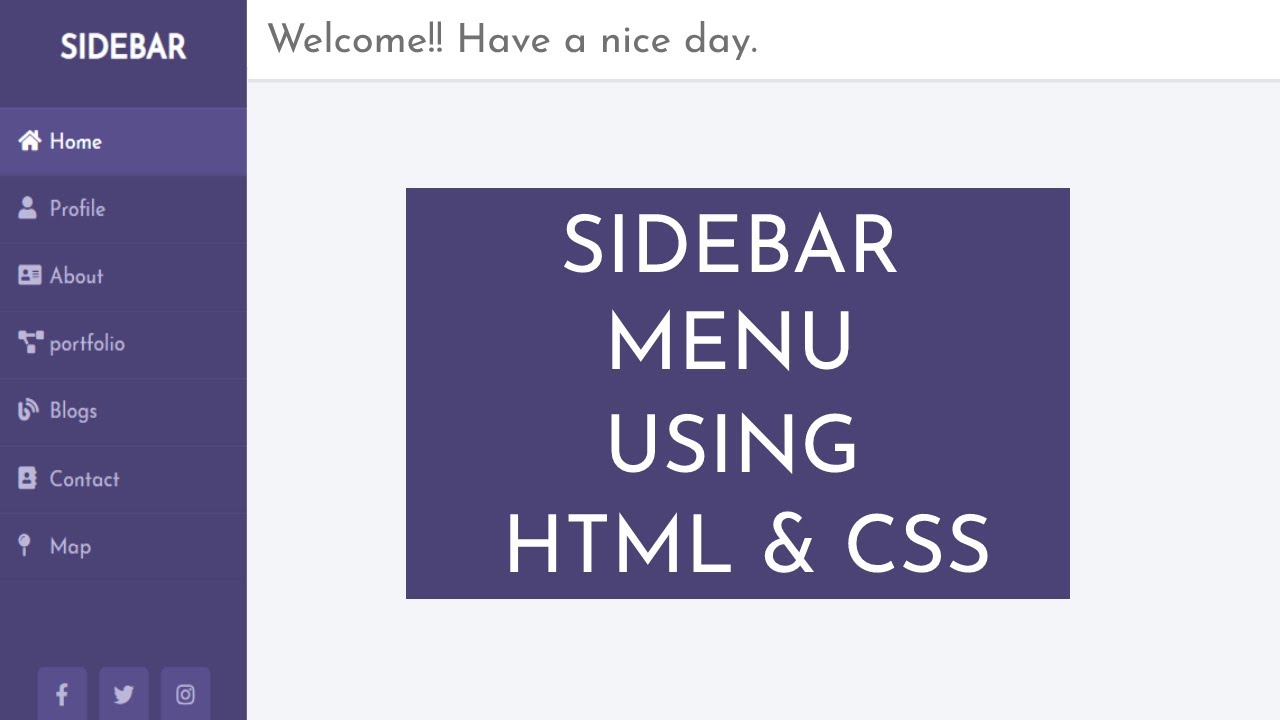The image captures a computer screen displaying a sidebar menu on a webpage. At the top of the screen, under a section labeled "Sidebar" in white text on a grayish-purple background, a vertical grayish-purple rectangle extends down the left side, serving as the sidebar. Within this sidebar, various interactive icons are listed sequentially. Each icon represents a different section: a house icon for "Home," a person icon for "Profile," a news article icon for "About," connected squares icon for "Portfolio," a bee icon with lines for "Blogs," an address book icon for "Contact," and a magnifying glass icon for "Map." At the very bottom of the sidebar, social media icons are displayed for Facebook, Twitter, and Instagram.

In the main content area of the screen, at the top center, a white rectangle bears the text "Welcome!! Have a nice day." Below this, a grayish box occupies the bottom part of the screen, with a central purplish box that reads "SIDEBAR MENU USING HTML AND CSS" in capital letters. This captures the essence of the webpage layout and the options available within the sidebar menu.